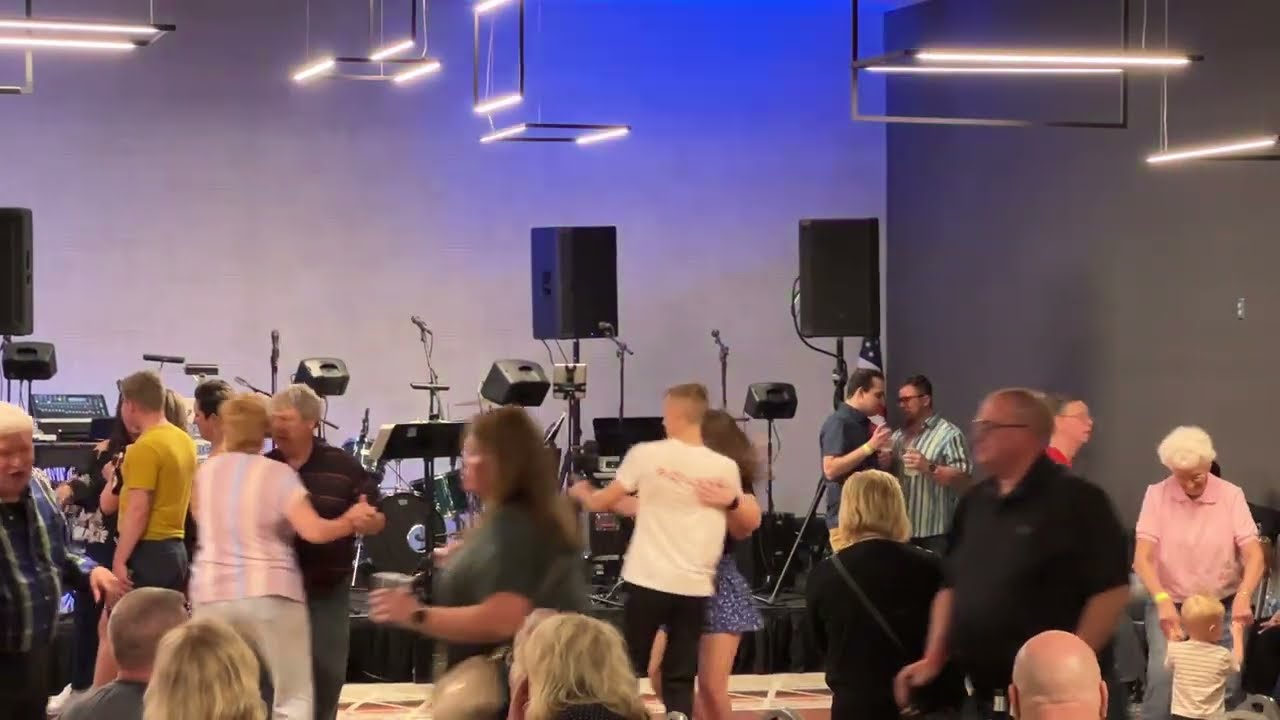The image appears to depict a lively event, potentially a wedding reception or party, set in a spacious venue with a stage. The stage, which stands slightly elevated, is equipped with a drum set, musical instruments, microphones, and tall speakers, but is currently empty of musicians. Fluorescent, geometric lighting fixtures are positioned above the stage, casting an even glow across the scene. In the foreground, people of various ages, dressed mostly in casual t-shirts and short-sleeved shirts, are dancing and mingling. A striking detail is an elderly woman with white hair in a pink shirt dancing joyfully with a young boy, around three years old, in the bottom right corner. Other noted individuals include a man in a black shirt, another person in a yellow t-shirt wandering about, and a couple comprising a man in a white shirt and a partner in a blue skirt. The room's walls are painted a light purple hue, adding to the festive ambiance. Despite the absence of live musicians, the presence of speakers and band equipment suggests that recorded music might be playing, keeping the crowd entertained and dancing.